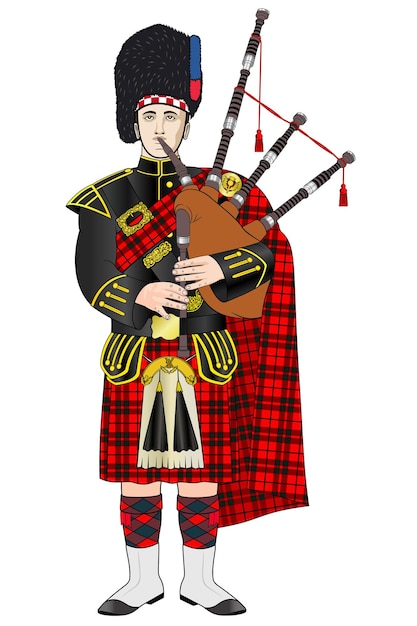The image is a detailed color illustration of a man playing the bagpipes. He is wearing a tall, black furry hat with a blue plume cascading down from one side, accented by a hint of red at the base. Around his forehead, a white and red checkered bandana is tied. The man is engaged in playing the bagpipes, with one of the pipes held to his mouth and his hands positioned on the lower part of the instrument. The bagpipes feature multiple tubes extending upwards. His attire includes a formal black jacket adorned with gold trims and yellow vertical striping on the cuffs. He is also draped in a red and black tartan kilt and cape. Adding to his traditional appearance, he wears matching red and black tartan knee socks and white shoes with black tips. A white sporran with two black tassels dangles from his waist, completing his outfit. Additionally, an elaborate red and black plaid completes the traditional Scottish ensemble, covering his right shoulder (from the viewer's left perspective). His eyes are slightly raised, looking towards the viewer.